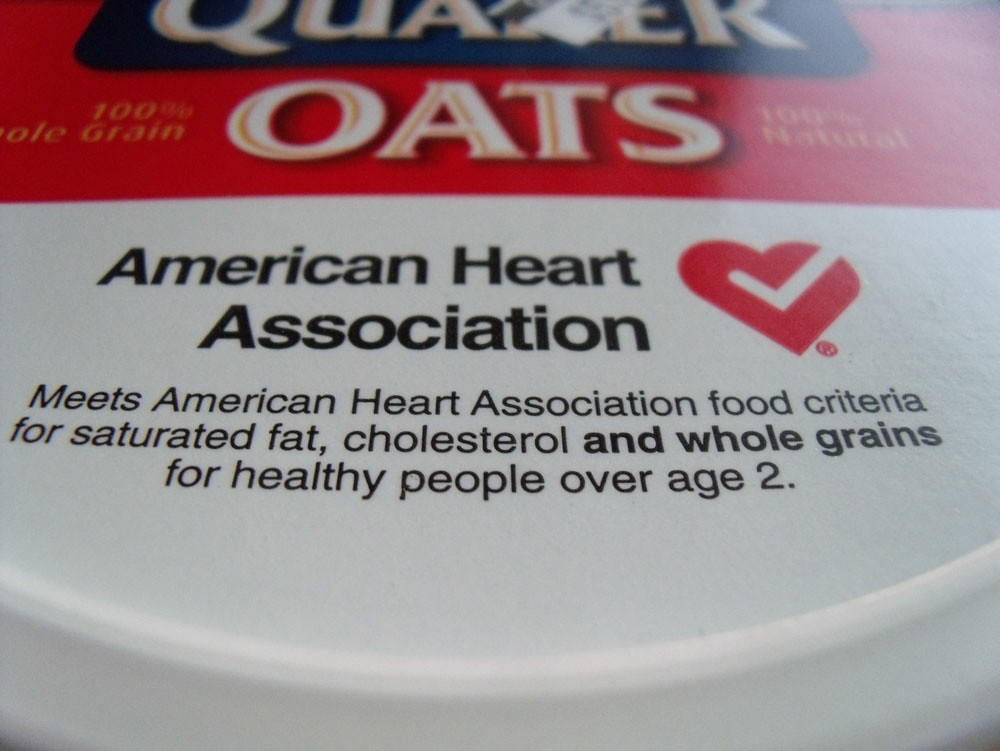The image showcases the top of a Quaker Oats container with distinct, colorful branding and health-related insignia. Dominating the top portion, the Quaker logo features white lettering on a blue background, although it is partially cut off. Below this, "Oats" is displayed in bold white letters on a red background. Prominent yellow text declares "100% Whole Grain" and "100% Natural," emphasizing the product’s health benefits. Centrally featured is the American Heart Association (AHA) logo, a red heart with a white checkmark, and accompanying text stating the product meets AHA criteria for saturated fat, cholesterol, and whole grains for individuals over two years old. The color scheme combines red, white, blue, yellow, and black text on a likely plastic lid, with the upper half in red and the bottom half in white.